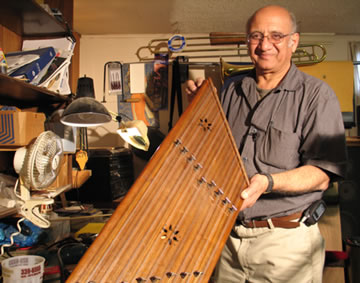In the photograph, a balding, middle-aged man with glasses stands proudly in a cluttered office or workshop. He is wearing a grey button-down shirt with a lot of items in the chest pocket, a brown leather belt, khaki pants, and a phone clipped to his belt. The man is smiling as he holds a wooden object with both hands. This object, possibly a musical instrument such as a harp or another string instrument, features rows of pegs, suggesting it might still need strings. The wooden device also has darker brown stripes and star-shaped cutouts. The background reveals a busy, slightly messy room with shelves holding scattered binders, folders, and brass instruments, including a trombone hanging on the wall, which reinforces the musical theme of the workshop. The room is well-lit, with beige walls, an overhead light, a fan, and a desk lamp visible in the scene.